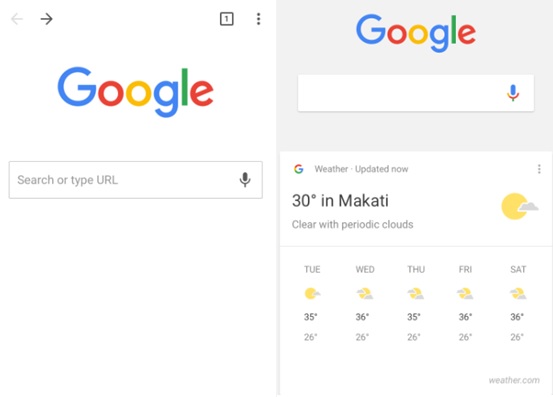The image features two separate screenshots side by side, displaying different states of the Google Search mobile app.

The left screenshot showcases a simple interface featuring the Google Search app in its default state. At the top of the window, there are forward and back navigation arrows, followed by a small outlined square with the number '1' centered in black. Adjacent to this square are three vertical dots represented by an ellipsis. Below this navigation bar, the iconic Google logo is prominently displayed with each letter in a distinct color: the 'G' in blue, the first 'O' in red, the second 'O' in yellow, the 'G' in blue, the 'L' in green, and the 'E' in red. Directly beneath the logo is a rectangular search field, prominently outlined, which bears the text "Search or type URL" in gray font. Positioned on the right within the search field is a small microphone icon, suggesting the option for voice search.

The right screenshot depicts an active search result in Google Search. At the top of this image is a gray rectangle housing the Google logo. Below it is the search field similar to the one in the left screenshot, but noticeably, the microphone icon at the right end of the field is now blue. The main content beneath this bar indicates a weather update for Makati. It reads, "Weather updated now: 30 degrees in Makati, clear with periodic clouds," accompanied by an icon of a sun partly obscured by a cloud. Further down, there is a five-day weather forecast, though specifics are not elaborated in the provided description.